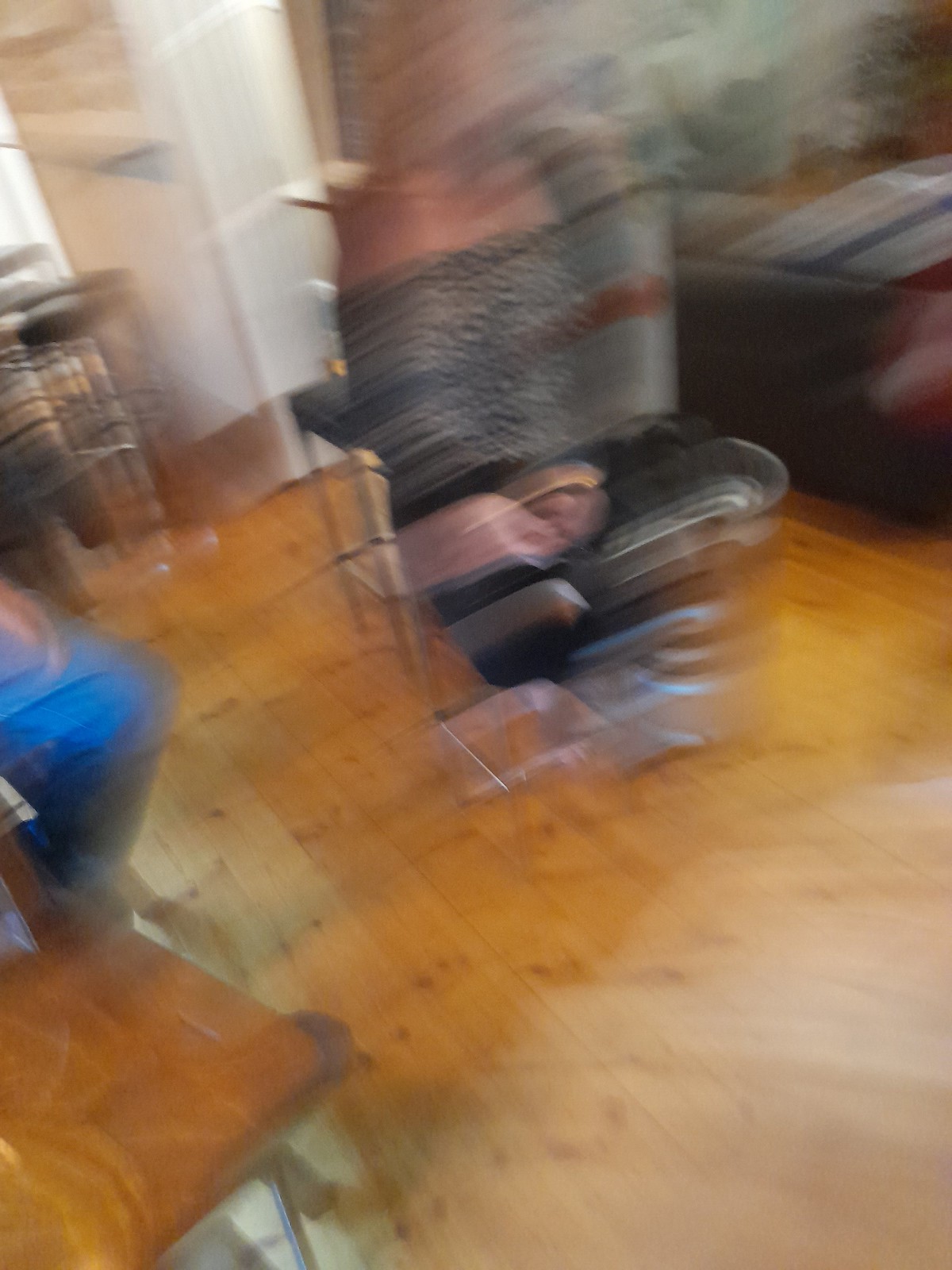The image portrays an extremely out-of-focus scene, likely of a living room. The floor is made of light brown hardwood, featuring diagonal lines running towards the bottom right. In the middle of the image, there's a person with white skin, possibly a woman with blondish hair falling to her neck. She’s clad in a black blouse adorned with white dots and black shoes. To the right of her, a blurry brown couch is visible, with what appears to be a bluish-white object on it. On the bottom left, there is an empty wooden chair slightly darker than the floor. The walls in the background are white, and on the left side, some blue item, possibly cloth on a table, is vaguely outlined.